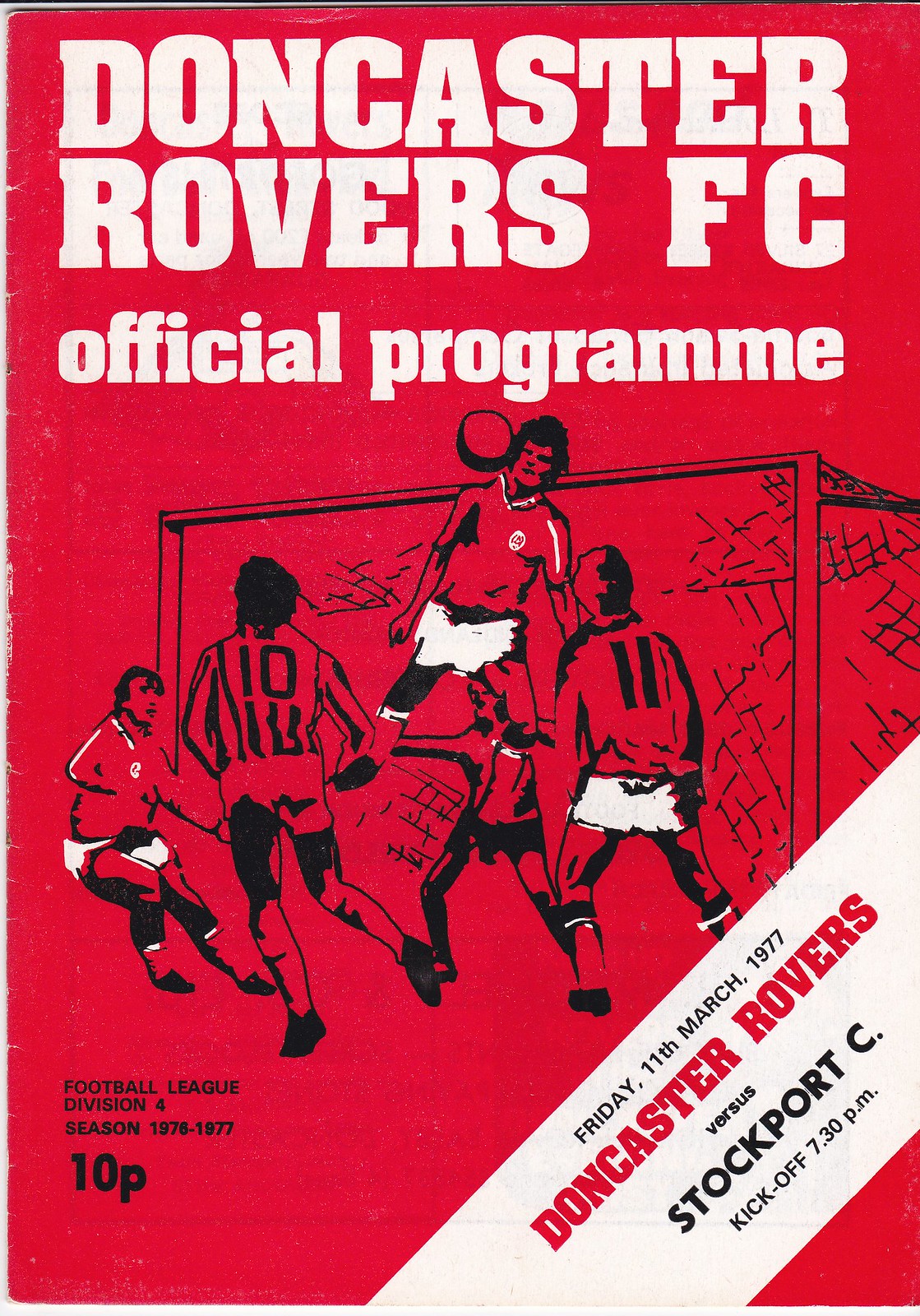This is an official program for the Doncaster Rovers Football Club, primarily featuring a rich red background with large white text. At the very top, "Doncaster Rovers FC" is prominently displayed, followed by the subtitle "Official Program". Below, it features the inscription, "Football League Division 4 Season 1976-77," along with the price, "10 P" in black text. The central artwork depicts five men playing football near the goal, with one player leaping high in the air to head the ball. Below this dynamic scene, it announces the match details: "Doncaster Rovers vs. Stockport C," set for Friday, 11th March 1977, with kickoff at 7.30 p.m.